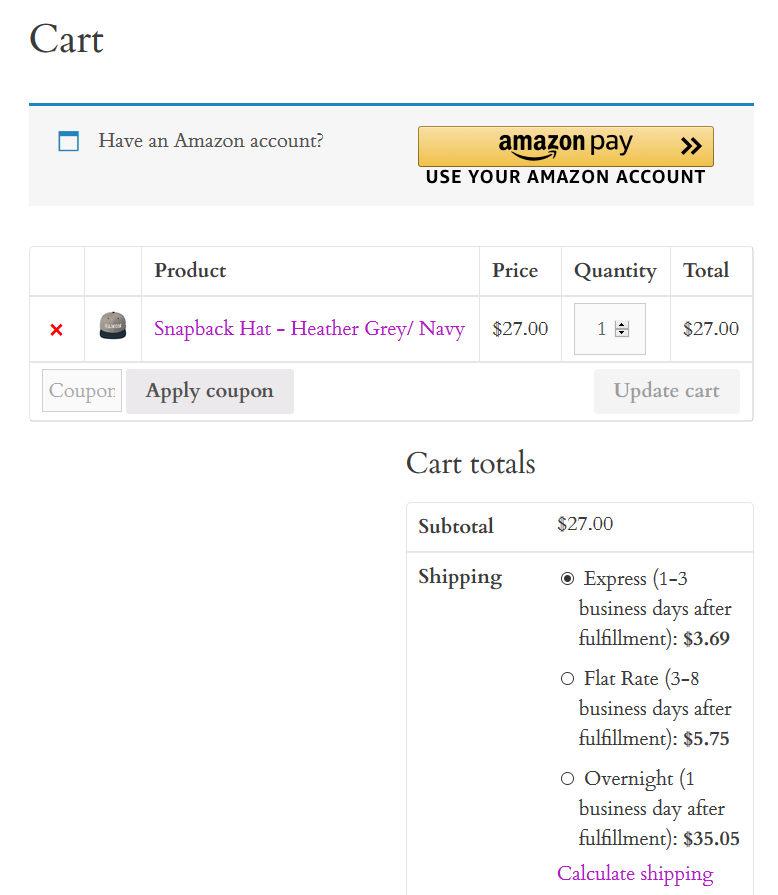The image depicts an Amazon checkout page. In the top left corner, a blue square box is prominently placed next to the text, "Have an Amazon account?" To the right of this, an orange rectangular box with the text "Amazon Pay" and the Amazon logo beneath it suggests a payment option via Amazon. Below this section, a call-to-action reads "Use your Amazon account," indicating a clickable button.

At the center of the page, inside a boxed area labeled "Product," there is a visual representation of the item being purchased—a Snapback Hat in Heather Gray/Navy. The product name is highlighted in pink text. Adjacent to the product image on the right, details such as the price ($27), quantity (1), and total cost ($27) are clearly displayed.

Towards the bottom left of this boxed area, there is a field for entering a coupon code next to the label "Coupon," accompanied by the "Apply Coupon" button. On the bottom right, an "Update Carts" button is available for modifications to the order.

Below this product information section, the "Cart Totals" area presents a summary: the "Subtotal" is listed as $27. Below that, various shipping options are detailed, including "Express," "Flat Rate," and "Overnight."

This detailed layout ensures that all pertinent information related to the purchase is visible and easily accessible for the user.